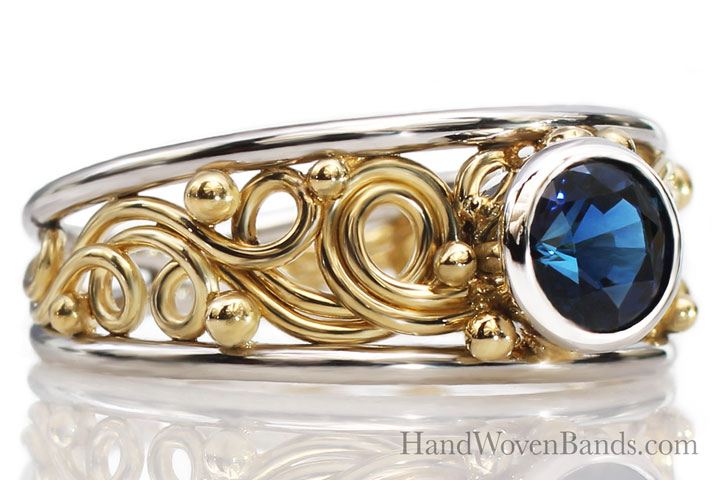This image is a high-resolution advertisement for handwovenbands.com, showcasing an intricate, ornate ring set against a stark white background. The main focus is a close-up of the ring, featuring a circular blue gemstone, likely a sapphire, set in a brilliant multi-faceted cut. This central gem is mounted in a circular silver setting that seamlessly blends into the ring’s design. The band itself is a striking combination of silver and gold: two silver bands are beautifully intertwined with swirly gold patterns, which are adorned with small gold balls. These delicate golden elements weave through the inner part of the band, creating an intricate and captivating design. The ring's reflective surface casts a subtle shadow underneath, adding depth and dimension to the photograph.